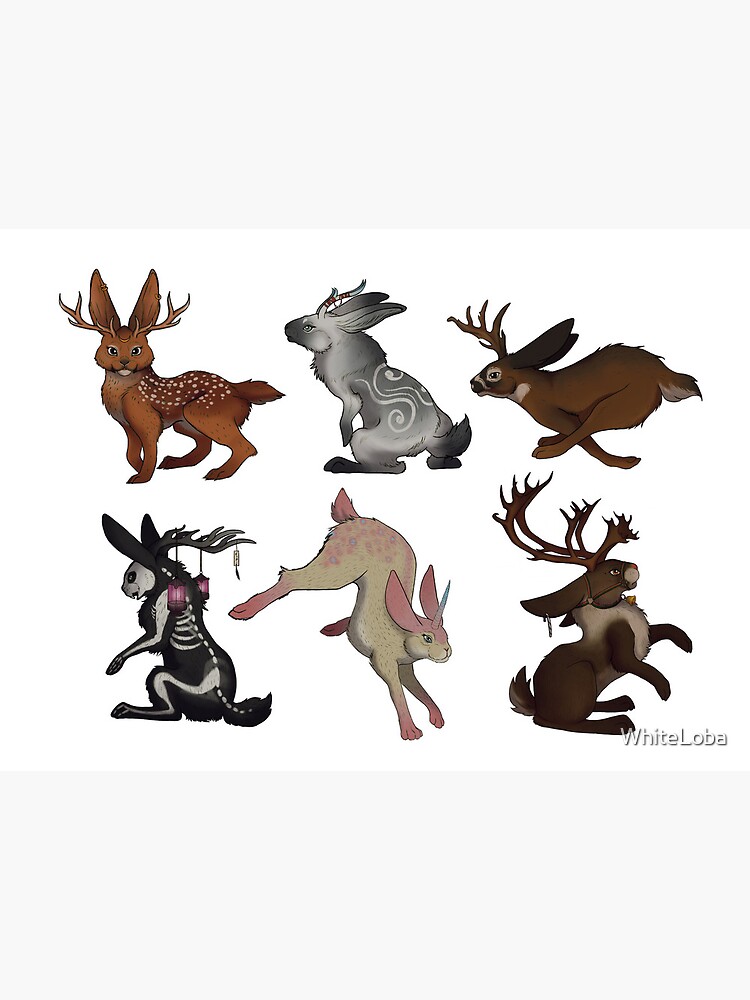The image is a compilation of clip art featuring six whimsical rabbits, each adorned with distinctive, fantastical features. These illustrations are organized in two rows of three. A watermark reading "White Loba" is present across the image.

1. The first rabbit, brown with deer-like antlers, has a spotted back mimicking that of a fawn and a gaze directed forward, blending characteristics of both a rabbit and a deer.
2. The second rabbit, depicted in gray tones, sports bifurcated antlers and intricate white spiral markings on its back, contributing to its mystical appearance.
3. The third rabbit is caught in mid-run, its posture dynamic with legs outstretched, featuring stag antlers, a dark brown coat, a black nose, and a white chest.
4. The fourth rabbit, black with a skeletal pattern, highlights its bones in a white outline. It has a skull-like face and adorns its black antlers with two hanging purple lanterns.
5. The fifth rabbit, in hues of pink and cream, showcases a more playful aesthetic with pink ears, a pink tail, pink socks on its feet, and a unicorn-like horn on its forehead.
6. The final rabbit, positioned upright on its hind legs with its front paws in the air, has a complete set of antlers and a bridle-like marking on its face, resembling a bucking horse.

Each rabbit's unique design intermixes realistic and fantastical elements, making the compilation appear ready for a quirky cartoon or fantasy movie.